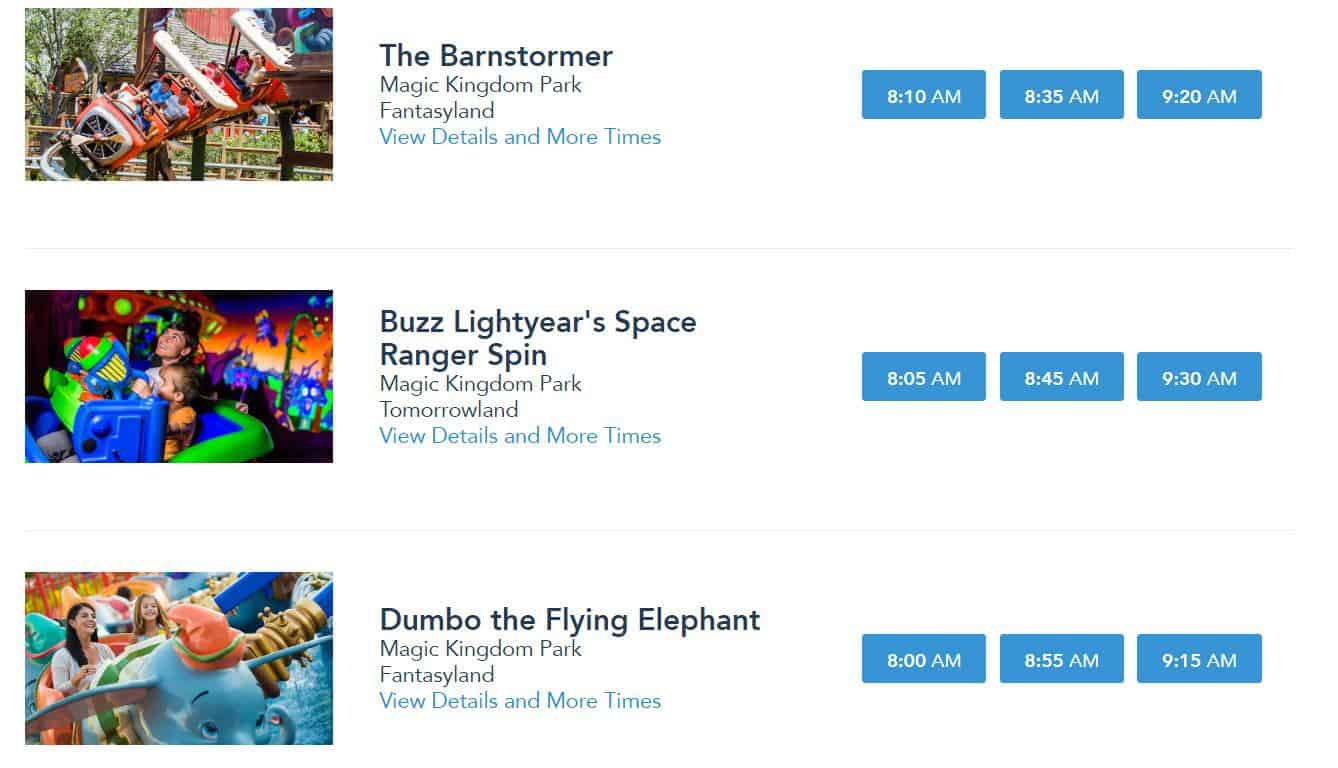The image is a screenshot from the Disney World app, displaying the reservation times for three popular attractions in Magic Kingdom Park: The Barnstormer, Buzz Lightyear's Space Ranger Spin, and Dumbo the Flying Elephant. Each attraction has a corresponding picture on the left side. The Barnstormer and Dumbo the Flying Elephant are located in Fantasyland, while Buzz Lightyear's Space Ranger Spin is in Tomorrowland. To the right of each ride are blue buttons indicating available reservation time slots. For The Barnstormer, the times listed are 8:10 AM, 8:35 AM, and 9:20 AM. Buzz Lightyear's Space Ranger Spin offers reservations at 8:05 AM, 8:45 AM, and 9:30 AM. Dumbo the Flying Elephant has time slots at 8:00 AM, 8:55 AM, and 9:15 AM.